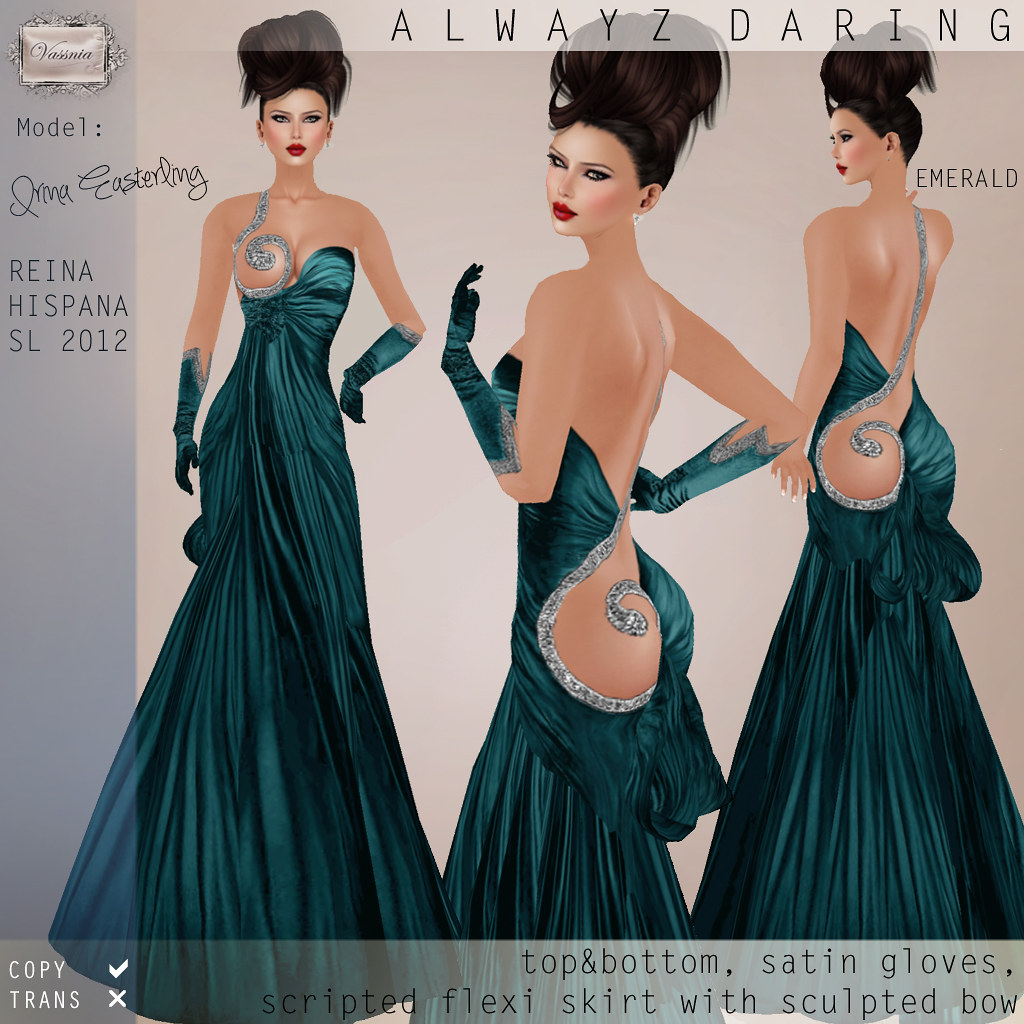This visually captivating color illustration, styled as a vintage magazine cover, features three different views of a digitally created woman in a dark green, sequin-embellished dress with matching ballroom gloves. Emphasizing her elegant silhouette, the images highlight intricate design elements of the dress, including a metallic swirl at the bust and a striking silver outline around the left hip and buttock. The model, with her dark black hair fashioned high atop her head and red lips accentuated by black eyeliner, exudes timeless glamour. 

In the leftmost image, she faces forward, her bright brown eyes and nearly exposed left breast captured in a poised stance. Her left arm is bent at the elbow, nearly level with her hip. The center image presents her from behind, as she glances seductively over her shoulder, showcasing the dress's back cut-out design. The rightmost view offers a detailed look at her back, with the word "Emerald" inscribed near her shoulder. Above the model's elegant form runs a transparent white banner that reads, "Always Daring," with a distinctive 'Z' at the end of 'Always.'

The upper left corner features a silver box labeled "Varienna," and underneath it, the word "Monocolon." Further down on the left, a signature lies underneath the model's name, Irma Easterling, alongside the label "Reina Hispania SL 2012." At the bottom, another subtle white line runs across with the text, "Copy," "Check," "Trans," and an 'X' mark. Detailed design notes list "Top and Bottom Satin Gloves," "Scripted Flexi Skirt with Sculptum Bow," underscoring the meticulous creation of this striking illustration.